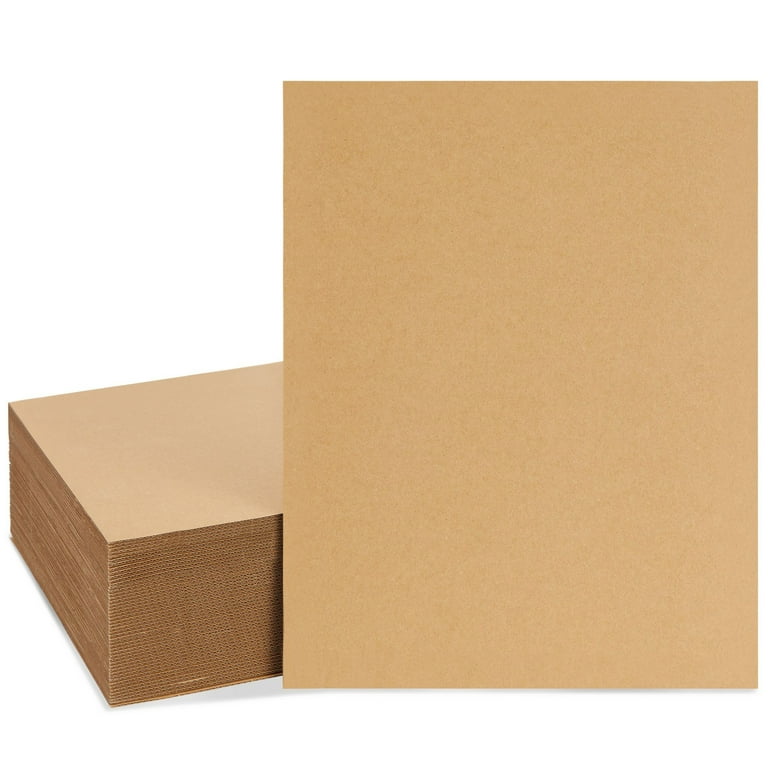This photograph features a stack of rectangular brown corrugated cardboard sheets set against a completely white background. The image is taken from an above angle, looking down upon the neat stack, with one individual sheet prominently displayed, leaning slightly towards the viewer. The cardboard, a standard tan brown color, varies subtly in shade from dark to light speckles, emphasizing its corrugated texture. The stack is composed of several dozen sheets, each resembling the size of a standard piece of printer paper. The detailed perspective showcases both the front and left side of the stacked cardboard, highlighting its layered edges and simple, utilitarian design.